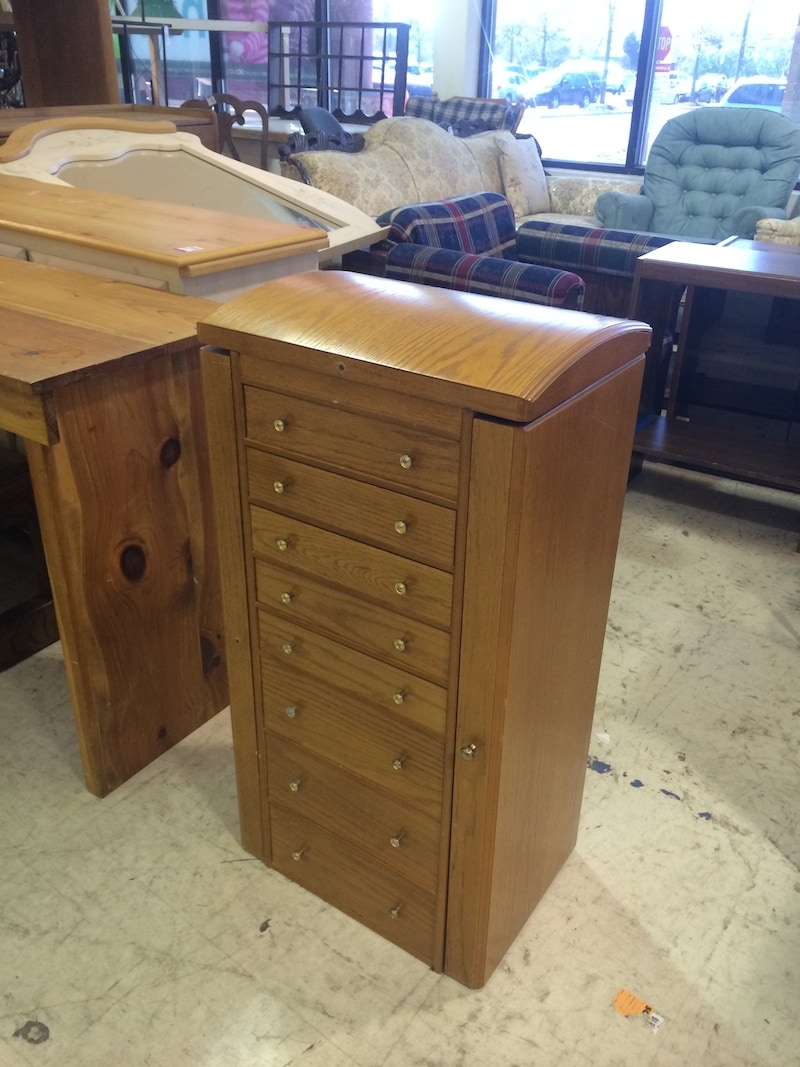This detailed photo captures the interior of a used furniture store, showcasing a variety of furniture items arranged across the showroom. Central to the image is a tall, narrow, light brown wooden dresser featuring eight drawers, each adorned with gold handles. The top five drawers are particularly shallow, while the bottom three offer slightly more depth. Additionally, a unique vertical pull-out drawer is visible on the right. Surrounding the dresser, a wealth of other furniture pieces are scattered throughout the showroom. To its immediate left, a gray and white sofa with a curved back and a single throw pillow can be seen. Positioned nearby is a bulky navy blue and red plaid chair. In front of this chair stands a wooden plant stand, ideal for placement behind a sofa. Towards the back of the scene, large windows reveal an outside view of a parking lot and street, where a stop sign is distinctly visible through one of the five windows. To the left of the dresser, partially visible, is a knotty pine piece that might be a desk. Behind this, another piece of furniture features a blonde wood top and a white base, possibly a dresser, complemented by a matching mirror above it. Beige flooring ties the scene together, grounding this eclectic collection of furnishings.